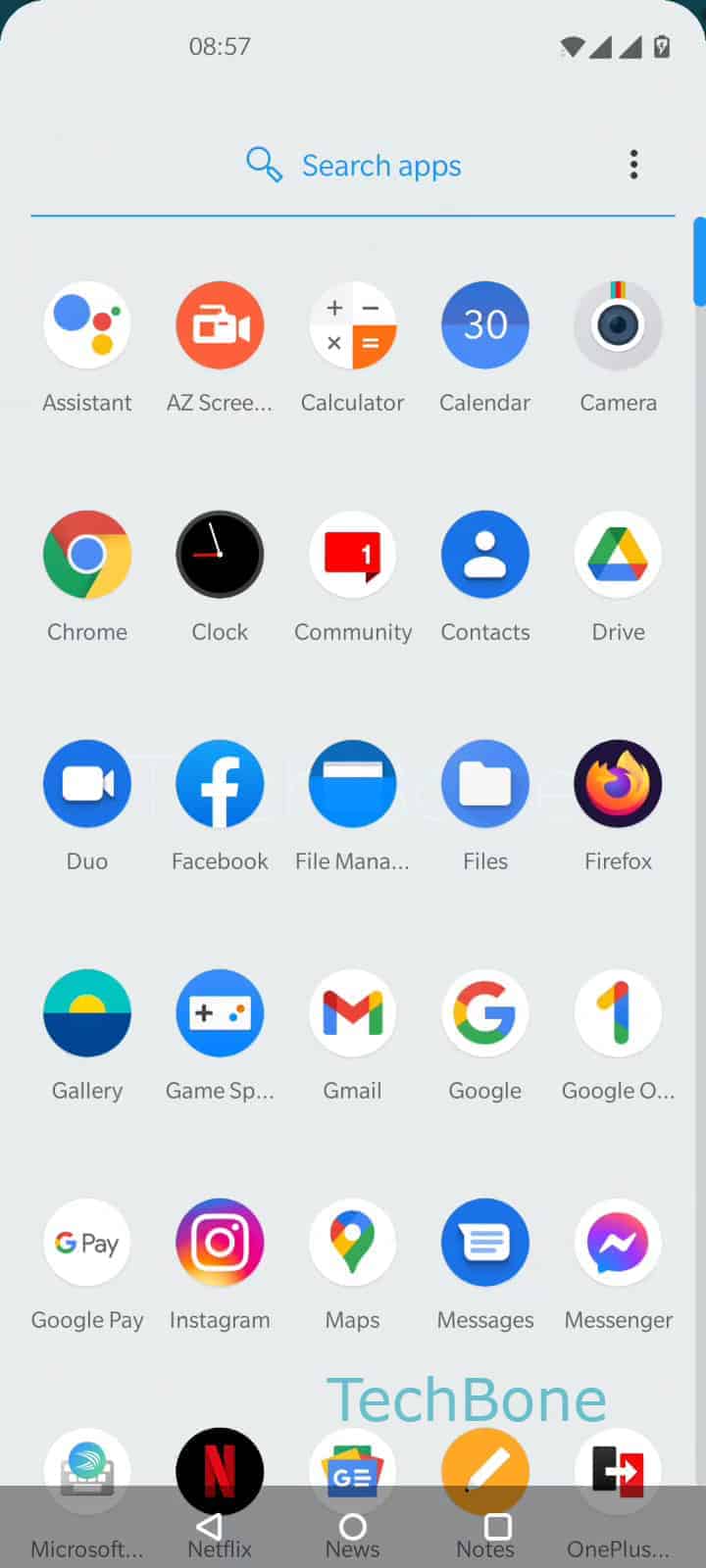This image captures a screenshot of a smartphone's home screen, notably densely populated with various apps arranged in a grid layout. At the top right corner, there's an icon indicating the phone is plugged in for charging. Adjacent to it are two phone signal strength icons, both fully filled in dark gray, signifying maximum signal strength. Further left, the Wi-Fi signal icon is also fully filled, denoting a strong Wi-Fi connection. In the middle left at the top, the time is displayed as 8:57. Directly below the time, there's a blue-text prompt, "Search apps," accompanied by a magnifying glass icon to its left. A horizontal blue line separates this search bar from the app grid below.

The app icons are organized in rows of five. The first row consists of Assistant, AZ Screen, Calculator, Calendar, and Camera. The second row includes Chrome, Clock, Community, Contacts, and Drive. The third row displays icons for Duo, Facebook, File Manager, Files, and Firefox. The fourth row features Gallery, Game, Gmail, Google, and Google One. The fifth row showcases Google Pay, Instagram, Maps, Messages, and Messenger. The final row at the very bottom includes Microsoft, Netflix, News, Notes, and OnePlus.

This detailed layout captures the diverse functionalities and tools accessible on the device, indicating a well-organized user interface designed for efficiency and easy navigation.